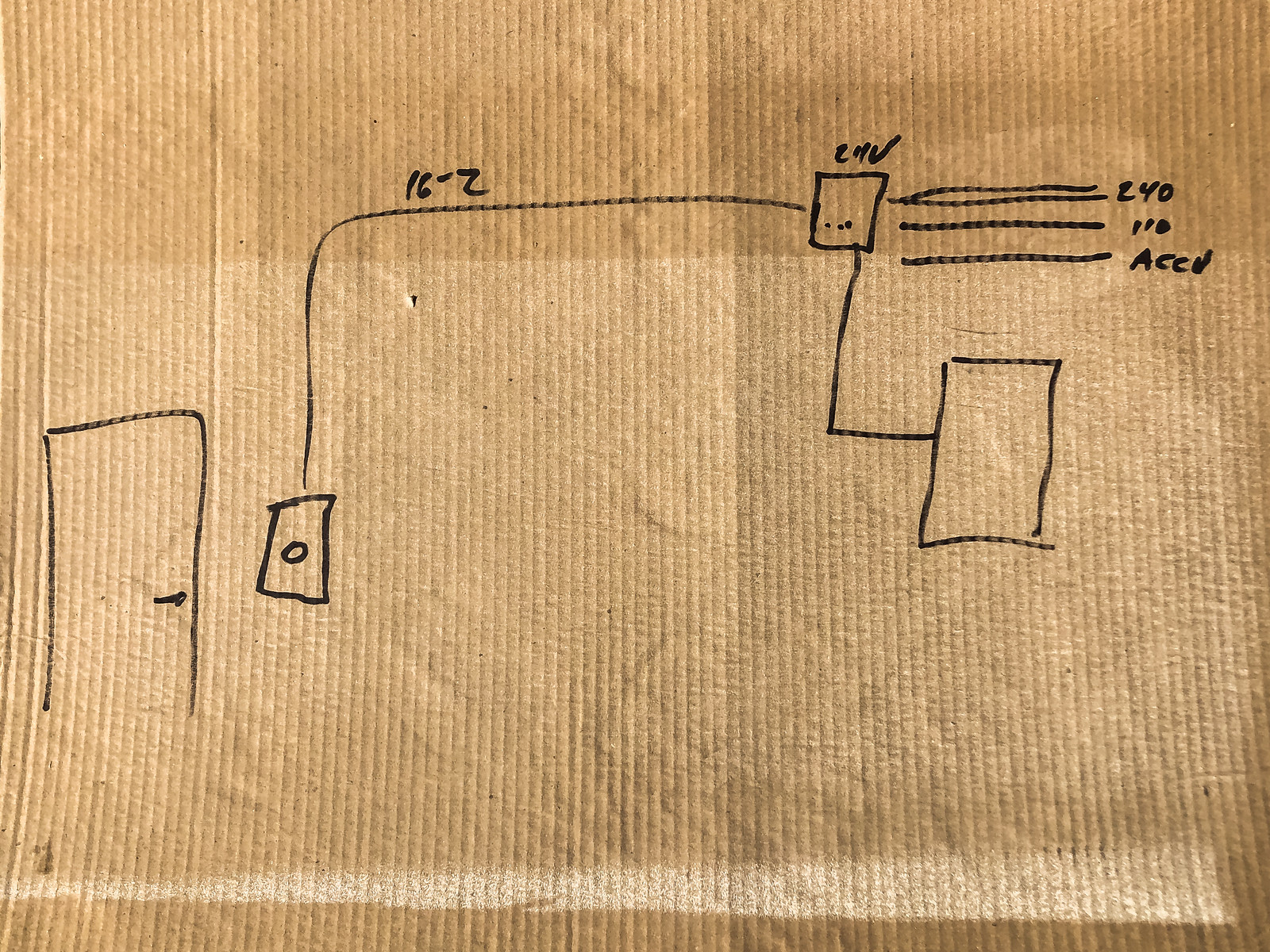The image appears to be a horizontal rectangular scan or photograph of a drawing, created on a brown cardboard-like surface that could either be actual cardboard or something similar with visible vertical ridges. The drawing itself seems to be crafted in black permanent marker, characterized by simple outlined shapes, lines, and numbers with minimal detail and no additional colors. 

On the extreme left of the image, there is a door depicted by three sides of a rectangle (left, top, and right) and a horizontal line indicating a door handle. Adjacent to the door on the right, a vertically oriented rectangle is drawn. This rectangle includes a circle in its center from which a line extends upwards, then turns 90 degrees to the right. At this junction, the notation "16-2" is written above the line. This line connects to a box positioned further up the page. 

Above this box, there are some indistinct markings. Extending horizontally from the right of the box are three or four parallel lines, which eventually lead to the text "240-110-ACCO" further to the right. From the previously mentioned box, another line extends downward, then turns to the right, leading to another vertical rectangle on the right side of the image.

Overall, the composition is a technical schematic or diagram rendered with basic line work and annotations on a textured brown background.